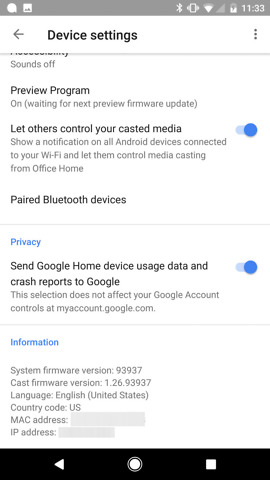The image shows a cell phone screen displaying specific device settings at 11:33 AM. The top section has a gray status bar indicating a strong connection, with various icons on the left side. Beneath the status bar, a navigation bar labeled "Device settings" in black stretches across the screen, with a back arrow pointing to the left.

The top portion of the settings menu is slightly cut off but includes the "Sounds off" option. Following this, there's a "Preview program" section. A highlighted blue option reads "Let others control your casted media," indicating it is enabled.

Further down, under "Paired Bluetooth devices," there's another light gray segment. Next, the "Privacy" section is highlighted in blue, offering the option to send Google Home device usage data and crash reports to Google. A blue circular information icon accompanies this option.

Additional information displayed includes "System firmware version" and "Cast firmware version" with corresponding numbers, "Country code" set to the US, and the language "English (United States)." The MAC and IP addresses are both grayed out, indicating they are not editable.

At the bottom of the screen, there is a thick black bar containing navigation buttons: a home button in the center, a square multitask button on the right, and a back arrow on the left.